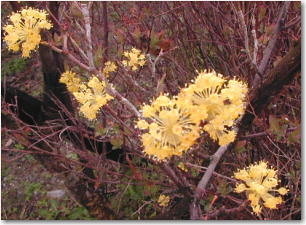This close-up image, taken outdoors likely during the fall or autumn season, captures a delicate scene under dim daylight. The primary focus is on a flowering bush with thin, tightly condensed stems that exhibit a purplish-red hue, while the thicker stems are grey. The bush is adorned with feathery, multi-petaled clusters of yellow blooms, varying in intensity from light to darker shades and displaying different stages of growth. Some of the flowers are notably large, situated around the center of the image, while others, particularly on the left, are considerably smaller, suggesting they are still growing. Complementing this scene, the foreground shows green leaves scattered among the grass and shrubbery, while the background features several nearly bare trees and a few with red leaves, reinforcing the autumnal setting. The right side of the photo possesses a shadow border, adding a subtle frame to this intricate natural tableau.